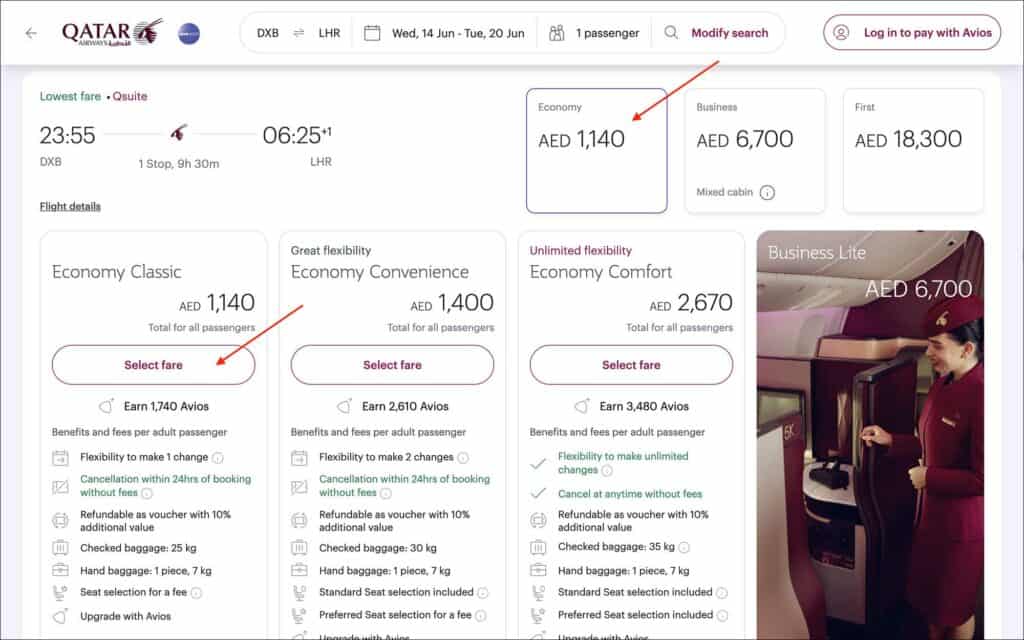This is a screenshot from Qatar Airlines' flight booking system. 

On the right side of the header, there's an icon featuring what appears to be an ibex or antelope within a circle. The header also includes the route marker "DXB LHR," referring to a flight from Dubai (DXB) to London Heathrow (LHR). Additionally, a calendar icon indicates the travel dates: from Wednesday, June 4th to Tuesday, June 20th, for one passenger, with an option to modify the search. To the far right of the header, there's a login option to pay with Avios points.

Below the header, the flight details are listed, displaying the lowest fare in Qsuite at AED 2,355. This flight departs at 23:55 from DXB, has one stop, and arrives at LHR at 06:25, with a total travel time of 9 hours and 30 minutes including a 6-hour layover. The booking options include Economy, Business, and First Class, with Economy being selected by default. The fares are displayed in AED: 1,140 for Economy, 6,700 for Business, and 18,300 for First Class.

Further into the details, three columns categorize Economy Class into Economy Basic, Economy Convenience, and Economy Comfort, with respective prices of AED 1,140, AED 1,400, and AED 2,670 per passenger. Each category explains the flexibility and cancellation options available. 

At the bottom of these columns are buttons to select the fare, styled with burgundy text within a white capsule. The Economy Basic fare button is highlighted with a red arrow, as is another section in the upper right corner of the interface, guiding the user's attention.

The entire layout is rich in text, providing detailed information about fare types, total cost for all passengers, and additional conditions related to flexibility and cancellation policies.